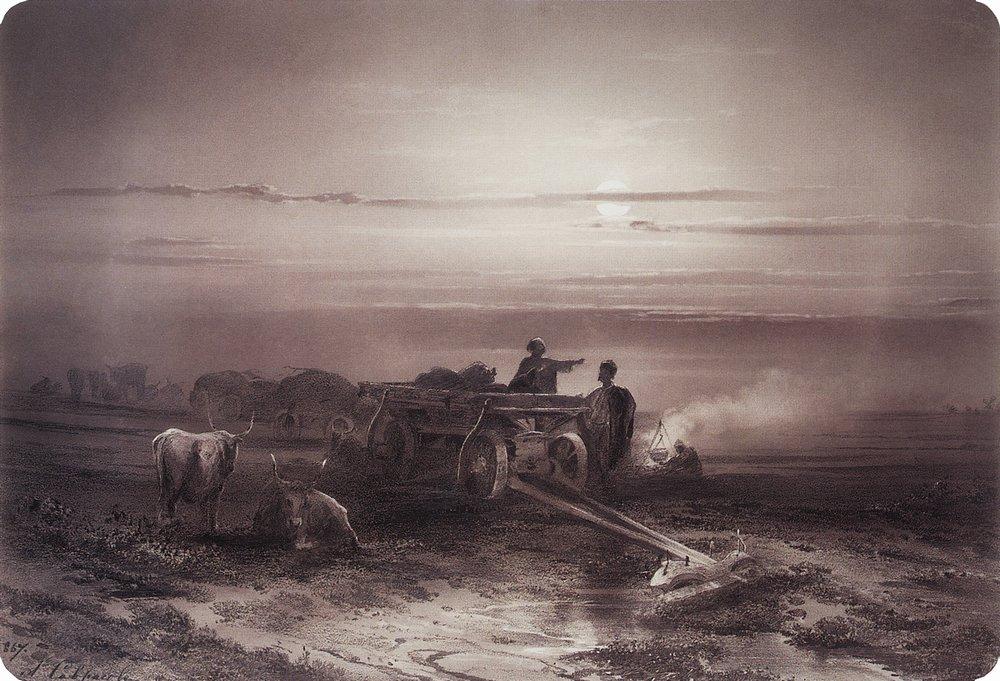This highly detailed black and white illustration captures a nighttime scene of a wagon train in a barren, muddy field. The dark sky above is strewn with clouds partially obscuring the moon. In the foreground, two long-horned cows are depicted, one standing and the other lying down on the muddy ground. At the center of the image, a wooden wagon loaded with several dark gray sacks stands prominently. Next to the wagon, a man gestures to the right while another man stands beside him, looking to the left. Behind them, a person tends to a kettle cooking over a small fire, seated on the ground. Multiple wagons are visible in the distance, further conveying the sense of a traveling group encamped for the night. The scene evokes a sense of rugged hardship and communal effort under the dim light of a cloud-streaked moonlit sky.